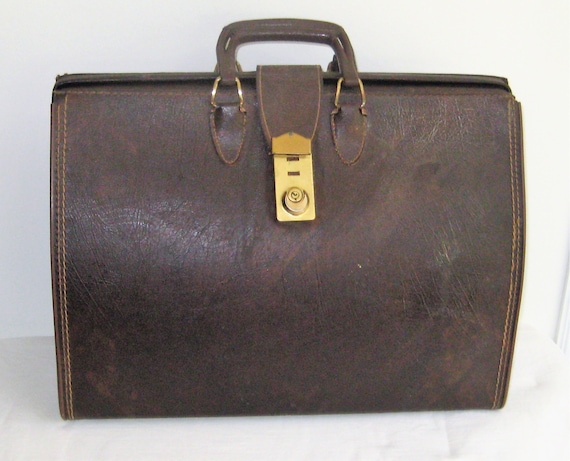This image showcases a large, brown leather bag with a slightly distressed finish, leaning against a light white wall. The rectangular, expandable bag has two short handles at the top, secured with brass loops and stitching visible on both sides. A brass locking system, including a buckle and a gold-colored plate, secures a leather strap that keeps the bag closed. The bag appears slightly bulging at the sides, indicating it may be holding items within. The leather has a subtle shine, particularly noticeable on the left side, and the background is an off-white color.